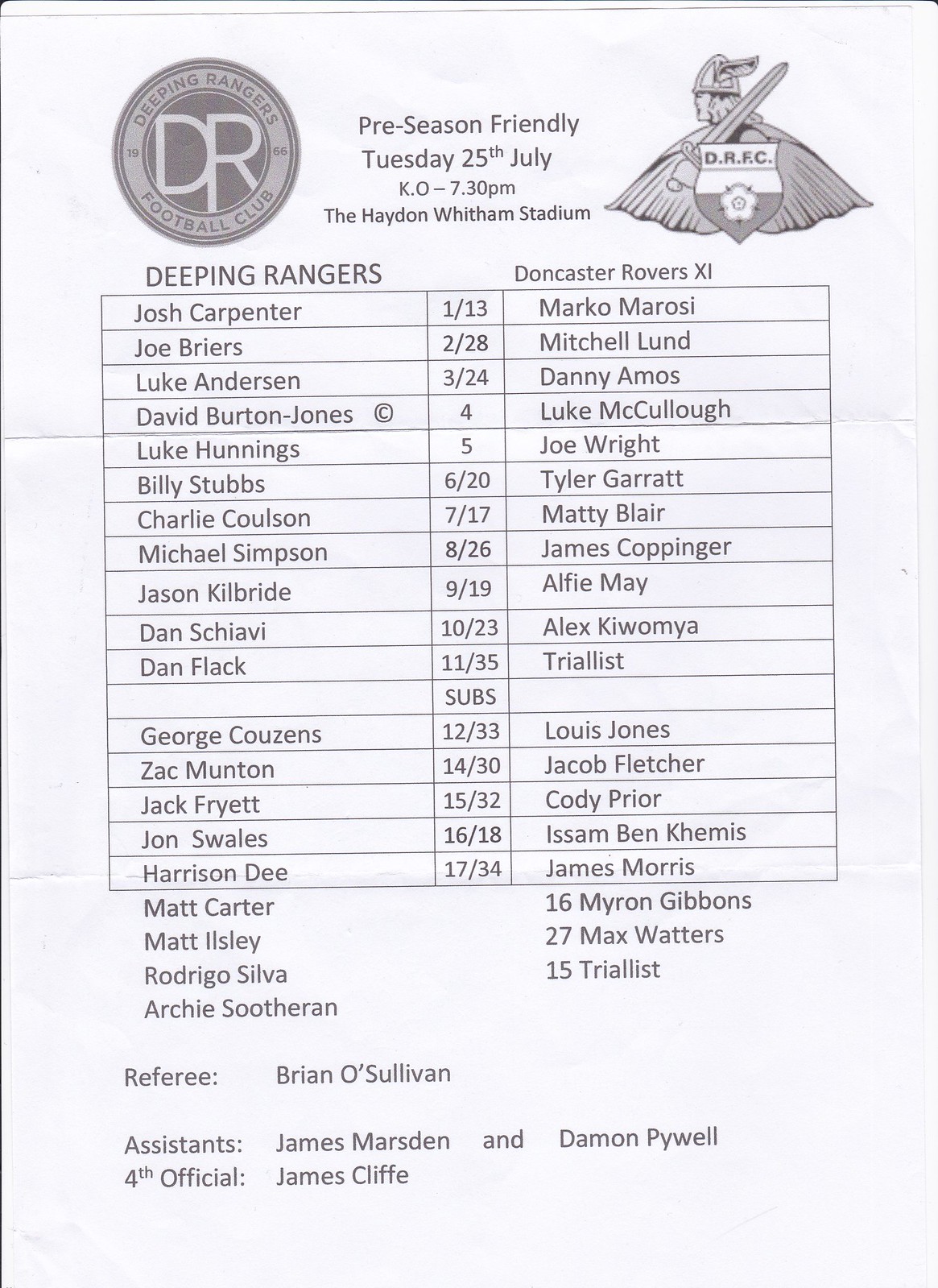This image is a comprehensive page from a soccer program for a pre-season friendly match on Tuesday, 25th of July, with a kickoff at 7:30 p.m. at Hayden-Whitman Stadium. The top of the page prominently displays the logos and emblems of the Deeping Rangers Football Club. In the top-right corner, there is an illustration of the team's mascot, a Viking with a helmet, holding a sword and shield. Adjacent to it is a circular emblem with "DR" in the center, surrounded by the words "Deeping Rangers Football Club."

Below the headers, the page details the lineups for the match between the Deeping Rangers and the Doncaster Rovers XI. The layout includes three columns: the left column lists the players for the Deeping Rangers, the right column lists the players for the Doncaster Rovers XI, and the center column displays jersey numbers, some separated by slashes indicating shared numbers between players.

Additionally, the program lists the substitutes, referencing numbers in the middle column. At the bottom, the referees are named, with Brian O'Sullivan as the main referee, James Marston and Damon Pyle as the assistants, and James Cliff as the fourth official. The information is designed to allow fans to identify the players on the field effectively.